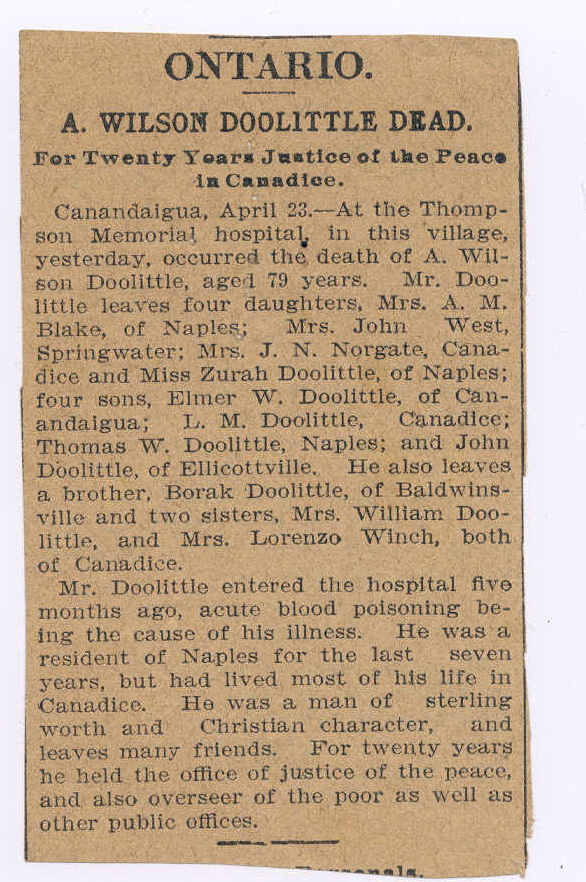The image depicts a vintage black-and-white newspaper clipping, meticulously cut out and centered against a gray or almost tan background. The clipping appears aged, with slightly brownish paper and black text alluding to its old-fashioned print. The article, an obituary, prominently features the word "ONTARIO" in bold at the top, followed by the headline, "A. Wilson Doolittle Dead for 20 Years, Justice of the Peace in Canadese." The main text is divided into two paragraphs. The first paragraph begins with "Kenan Daigua, April 23, at the Thompson Memorial Hospital," and recounts the recent death of A. Wilson Doolittle, aged 79, highlighting his legacy and family. He leaves behind four daughters: Ms. A. Blake of Naples, Ms. John West of Springford, Ms. Jane Norgate of Canadese, and Ms. Zora Doolittle of Naples, along with four sons and additional relatives, including a brother and two sisters (names not listed). The second paragraph notes that Mr. Doolittle had been hospitalized for five months due to acute blood poisoning, which ultimately caused his demise. The overall style is evocative of an early 20th-century newspaper, capturing the somber reflection on Mr. Doolittle's life and contributions.